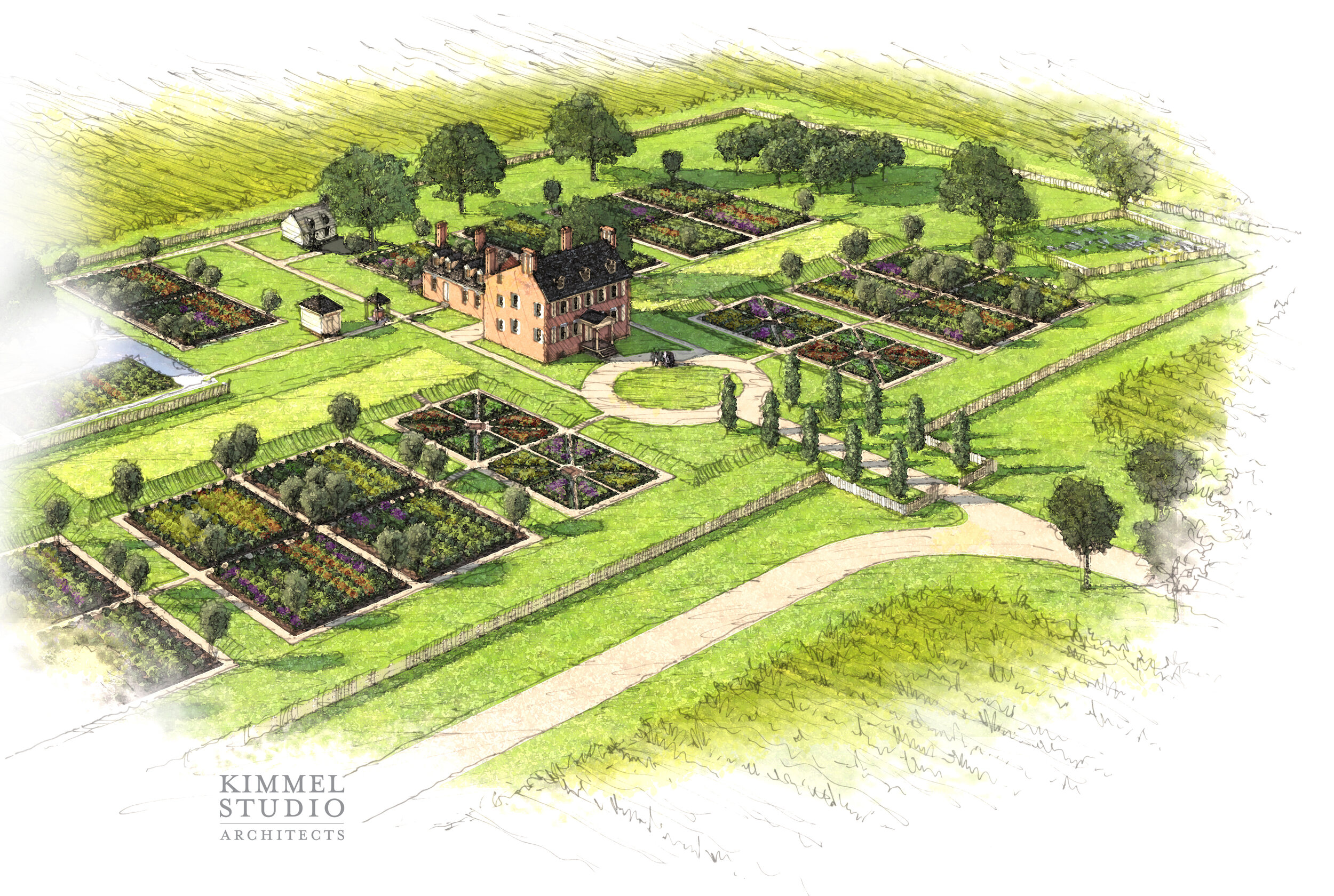The image depicts a meticulously hand-drawn layout of a planned landscape development, likely for a wealthy client, authored by Kimmel Studio Architects, as indicated by the label at the bottom left. Central to the design is an expansive colonial-style, three-story estate boasting ample windows, three chimneys, and a distinct circular driveway at the front. This grand house is surrounded by a balanced, symmetrical arrangement of gardens and pathways, suggesting a carefully curated landscape. Flanking this main structure are additional buildings, including a smaller two-story house with two chimneys, a barn-like shed, and another diminutive house on the periphery. The estate sits within a picturesque, English countryside-inspired setting, featuring tall trees lining the driveway and extensive garden plots. The overall composition, rendered possibly with colored pencils, exudes a sense of opulence akin to that found in affluent rural estates.